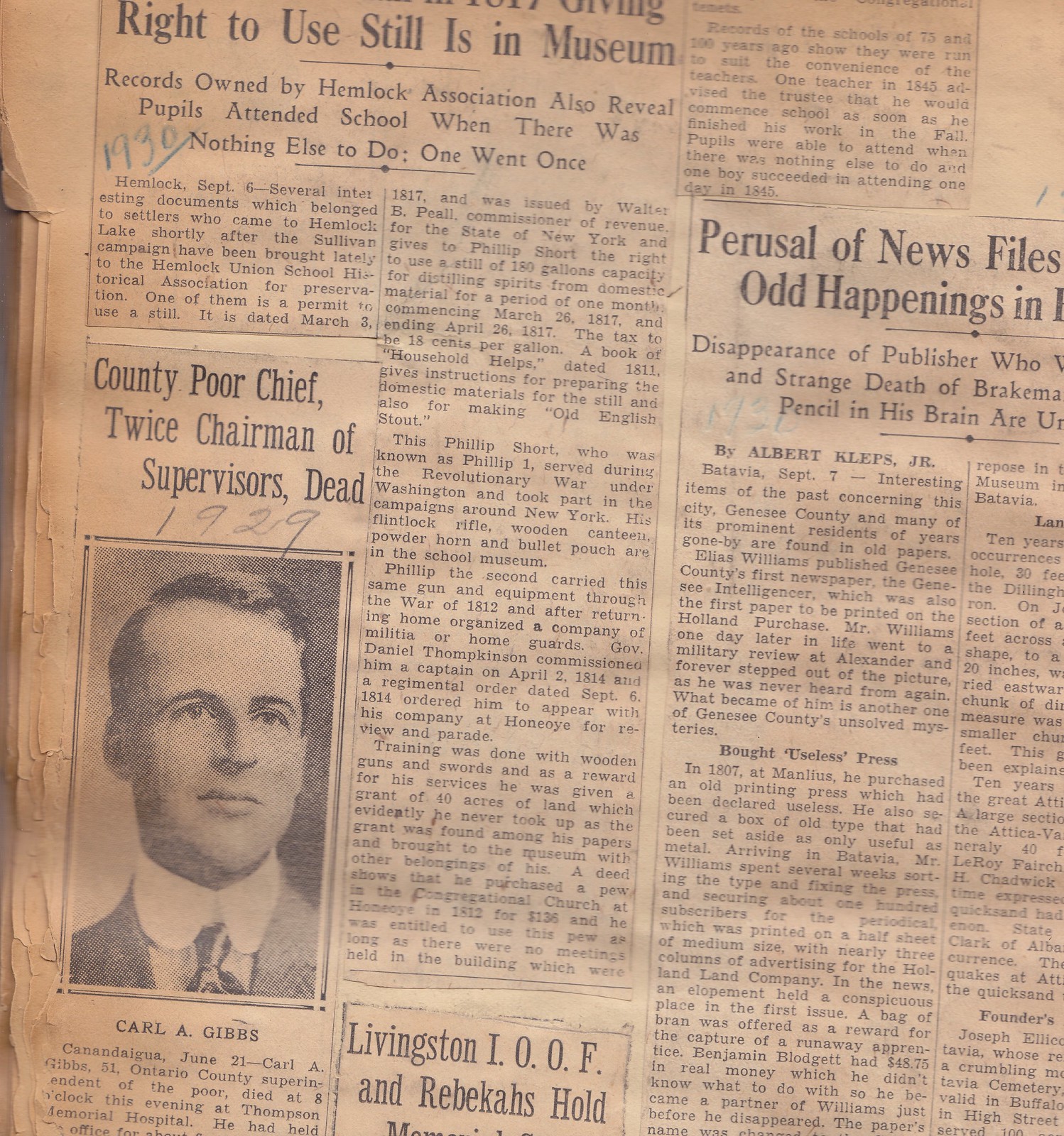This aged newspaper page, yellowed over time, features a collection of articles, prominently highlighting the passing of Carl A. Gibbs. At the bottom of the page is a black and white photograph of Carl A. Gibbs, identified underneath the image. Gibbs, a Caucasian man with short hair, is depicted wearing a suit and tie. The surrounding text above and below his image states, "County Board Chief, Twice Chairman of Supervisors Dead." Beneath the caption, someone has handwritten "1929" in pencil. Additional handwritten notes in green pencil mark the year "1930" next to another article. The headlines around the paper are partially legible, with one at the top reading "Wright U Still is a Museum," and "Records Owned by the Hemlock Association Also Revealed Pupils Attended School When There Was Nothing Else to Do." On the right-hand side, overlapping articles include partial headlines such as "Perusal News Files" and "Happenings in." This layered composition of historical articles and handwritten annotations creates a snapshot of a bygone era, emphasizing the legacy of Carl A. Gibbs.